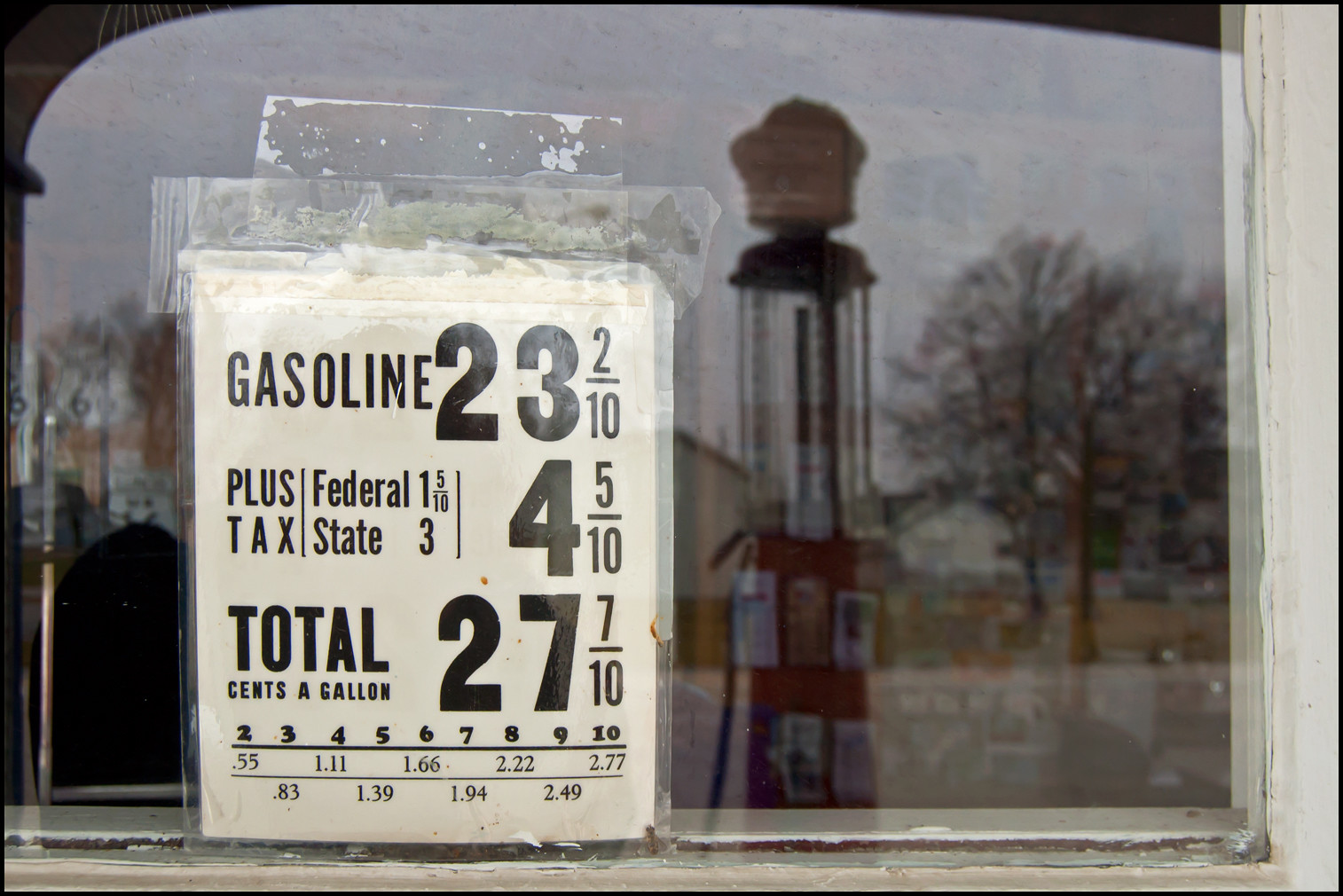The image in question appears to be a vintage photograph featuring an old gasoline pump from the late 1920s or early 1930s, set against a rural backdrop with houses and trees, and a couple of distant cars. The gasoline pump is prominently displayed with a laminated white sign taped to the forefront. The sign, showing signs of age and covered with clear tape, provides detailed pricing information in bold black lettering: "Gasoline, 23.2 cents per gallon, plus federal tax of 1.5 cents and state tax of 3 cents, totaling 4.5 cents in tax, for an overall price of 27.7 cents per gallon." The bottom of the sign also features a series of numbers and decimals, including sequences such as 2345678910, followed by .55, 1.11, 1.66, 2.22, 2.27, and below that .83, 1.39, 1.94, and 2.49. These additional numbers are not immediately clear in meaning but are likely related to pricing or other transactional details. The reflection in the glass of the window where the sign is taped captures more elements of the surroundings, including white and tan houses with black roofs, various trees, and some green and yellow grass. The photograph seems to capture a blend of historical context with a modern glimpse, indicating it was taken recently at an antique site.